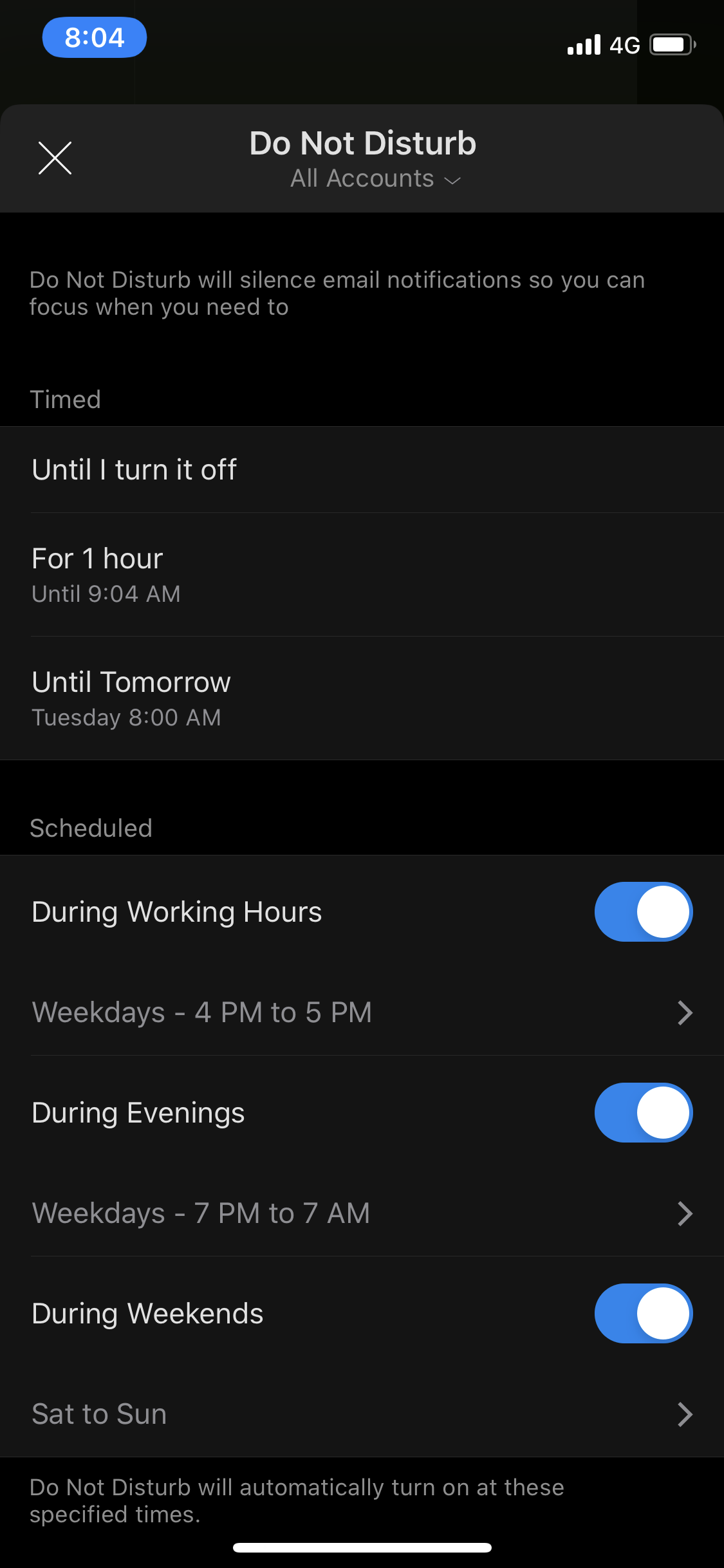Screenshot of a smartphone displaying the Do Not Disturb settings. The time is 8:04 AM, indicated on the screen within a blue, slightly oblong oval. The phone shows 4G network coverage and is currently set to Do Not Disturb mode for all accounts. A message explains that email notifications will be silenced to help with focus. The Do Not Disturb mode is scheduled to last for one hour, specifically until 9:04 AM, and is also set to continue until the next day, Tuesday at 8:00 AM. 

Scheduled timings for Do Not Disturb are detailed as follows:
- Weekdays from 4:00 PM to 5:00 PM.
- Weekday evenings from 7:00 PM to 7:00 AM.
- Entire weekends from Saturday to Sunday.

Do Not Disturb mode is also configured to turn on automatically at these specified times. The multitude of active periods suggests that the owner might be trying to minimize interruptions, possibly indicating this is a business phone or that they are on vacation. Buttons and sliders for customization are clearly shown, likely allowing further adjustment to these settings.